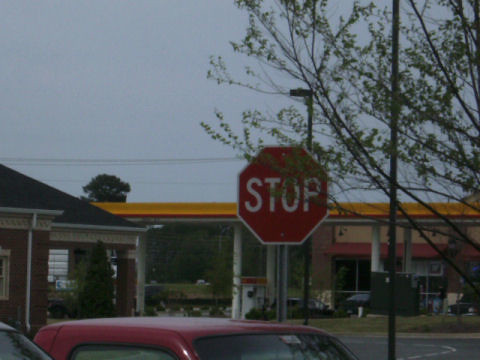In this photograph, the focal point is a red and white American stop sign positioned slightly right of center, partially obscured by thin green tree branches and shrubbery. Below the stop sign, the roof of a dark red vehicle is visible, suggesting it might be a truck, along with the corner of a silver-colored car. The scene appears to be set in a town's center, with the stop sign situated in the parking lot of a business that might be a bank, evident from the brown and white building to the left, featuring a drive-thru area and a black roof. Behind the stop sign is a paved road leading to a Shell gas station, identifiable by its distinctive yellow and red awning and white poles. Above the gas station, power lines stretch across a grayish-blue sky, indicating it could be late evening.